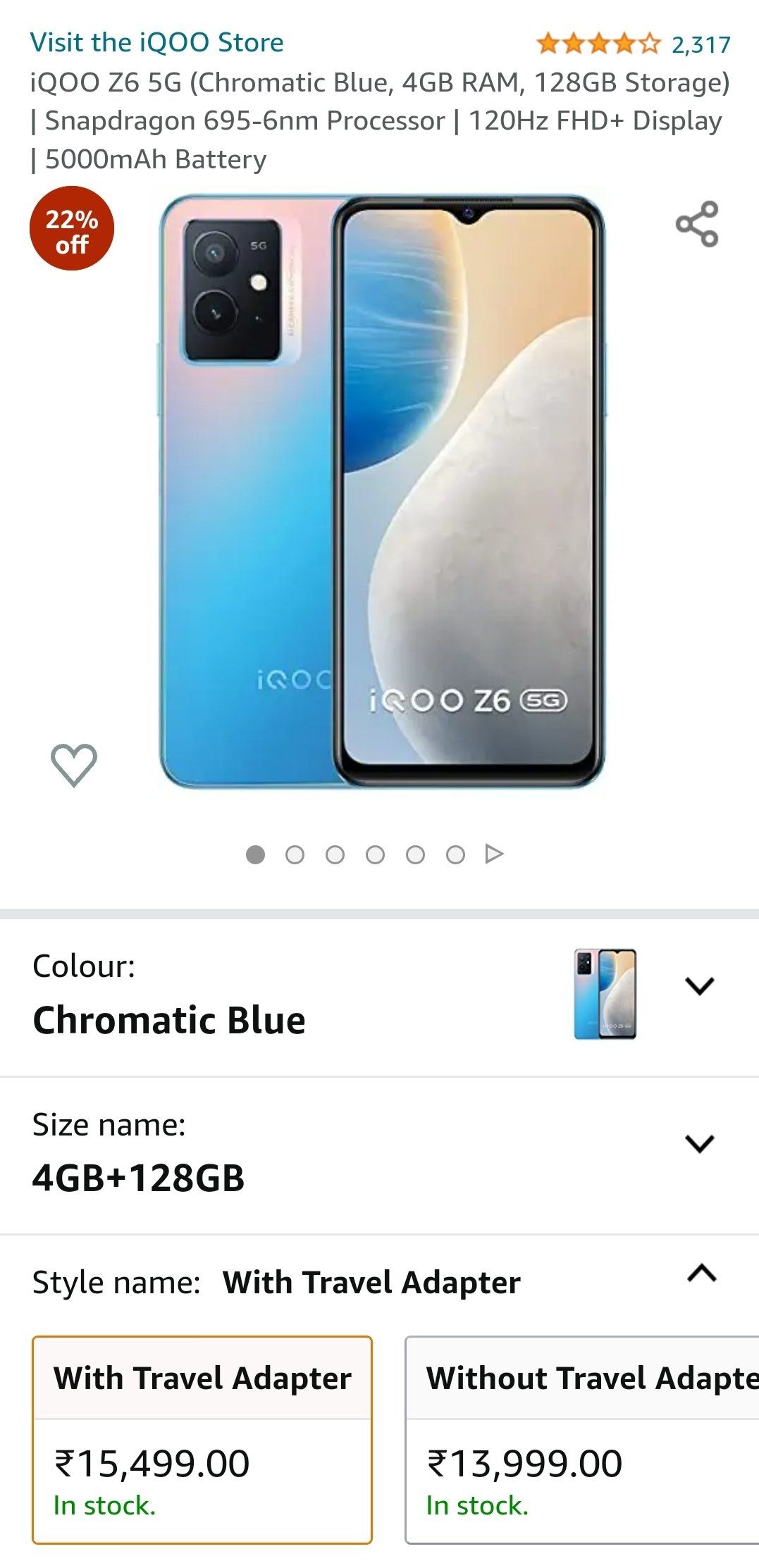Screenshot of an Amazon product page for the "IQOO Z6 5G" smartphone:

- **Product Name:** IQOO Z6 5G (Chromatic Blue, 4GB RAM, 128GB Storage)
- **Features:**
  - Snapdragon 695 6nm processor
  - 120Hz FHD+ display
  - 5000mAh battery
- **Top Left:** “Visit the IQOO Store” link
- **Top Right:** 4 out of 5 star rating, with 2317 reviews (typical orange star rating system used by Amazon)
- **Style Options:** Comes with or without a travel adapter
  - **With Adapter:** 15,000 (currency not specified, assumed to be in local currency)
  - **Without Adapter:** 13,000 (currency not specified, assumed to be in local currency)
  
The product page’s layout, including the text style and rating system, is identical to Amazon’s format. The chosen product variant is the Chromatic Blue color with 4GB RAM and 128GB storage capacity.